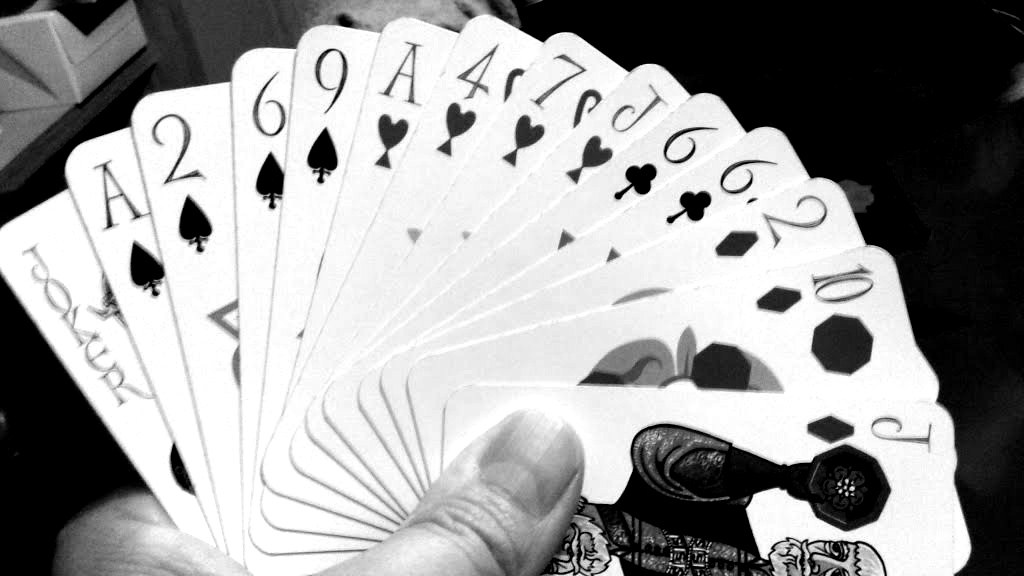In this striking black-and-white image, we see a Point of View (POV) perspective of a magician's left hand gracefully fanning out a sequence of 14 unconventional playing cards. The fan-like arrangement allows all the cards to be partially visible, showcasing an intriguing mix of suits and ranks. The cards are white but bear unique design and animation styles that differ from traditional playing cards. Among the visible cards, we have the Joker, Ace of Spades, Two of Spades, Six of Spades, Nine of Spades, Ace of Hearts, Four of Hearts, Seven of Hearts, Jack of Hearts, Six of Clubs, Two of Diamonds, Ten of Diamonds, and Jack of Diamonds. The Jack of Diamonds, with its distinct animation, stands out prominently, while the rest overlap to create an intricate, mesmerizing display. The blurry and indistinct background keeps the focus solely on the cards, enhancing the mystique and allure of the magician's artful arrangement.